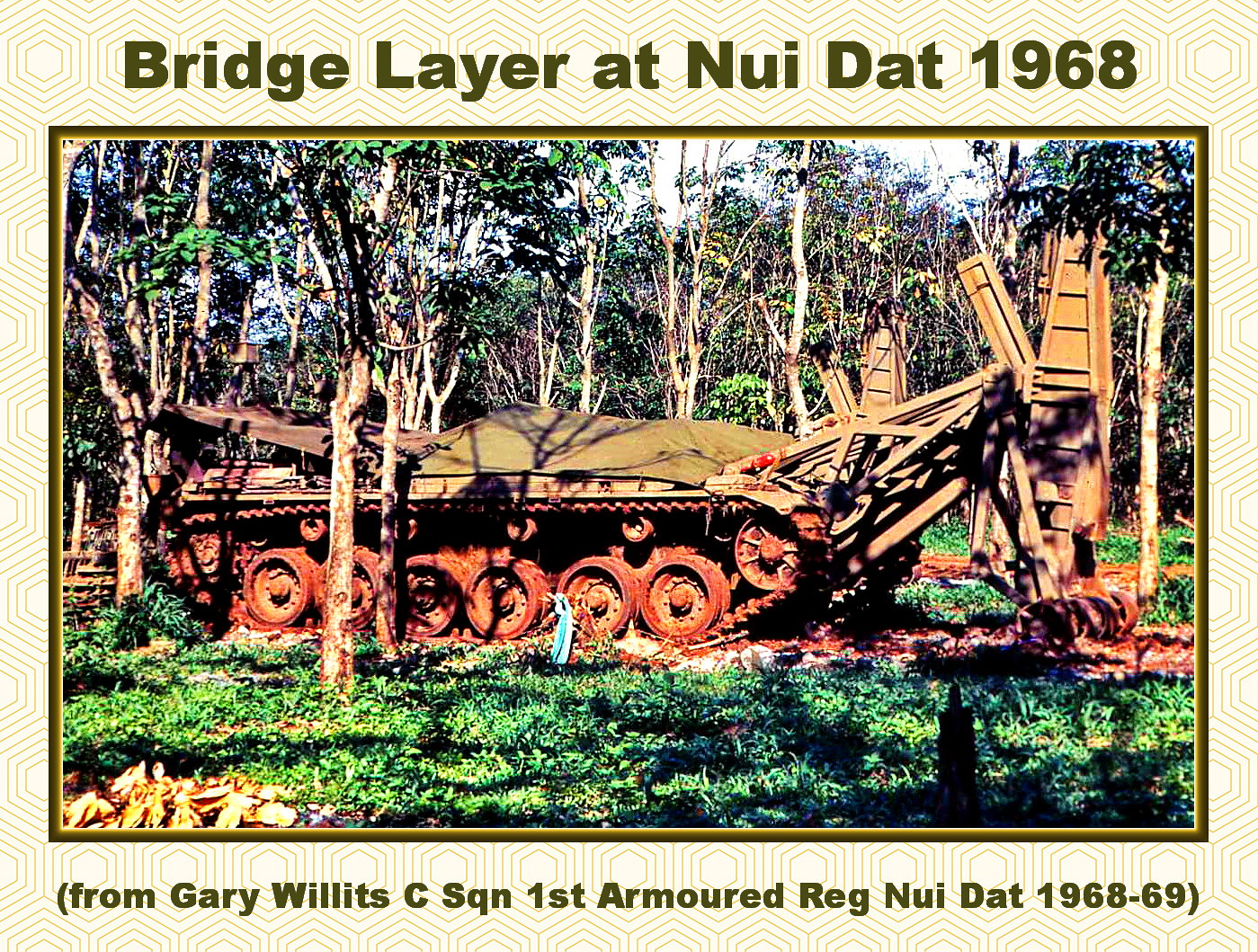This photograph, bordered by a light tan frame adorned with hexagonal patterns, features a rusted, Vietnam War-era bridge layer tank, captured in a jungle setting at Nui Dat in 1968. The caption at the top reads "Bridge Layer at Nui Dat, 1968," with an additional note at the bottom stating, "From Gary Willett, C-Squadron, First Armored Regiment, Nui Dat, 1968-69." The tank, used primarily by the Army Corps of Engineers to lay down bridges for other vehicles to cross, is adorned with deteriorating wheels and tracks, and appears to be partially covered by a tattered tarp. Nestled amongst green ivy and thin, spindly tree trunks, it seems to have collided with a structure, causing debris around it. The photograph also highlights a crane-like machinery attached to the tank, indicative of its specialized bridge-laying function.